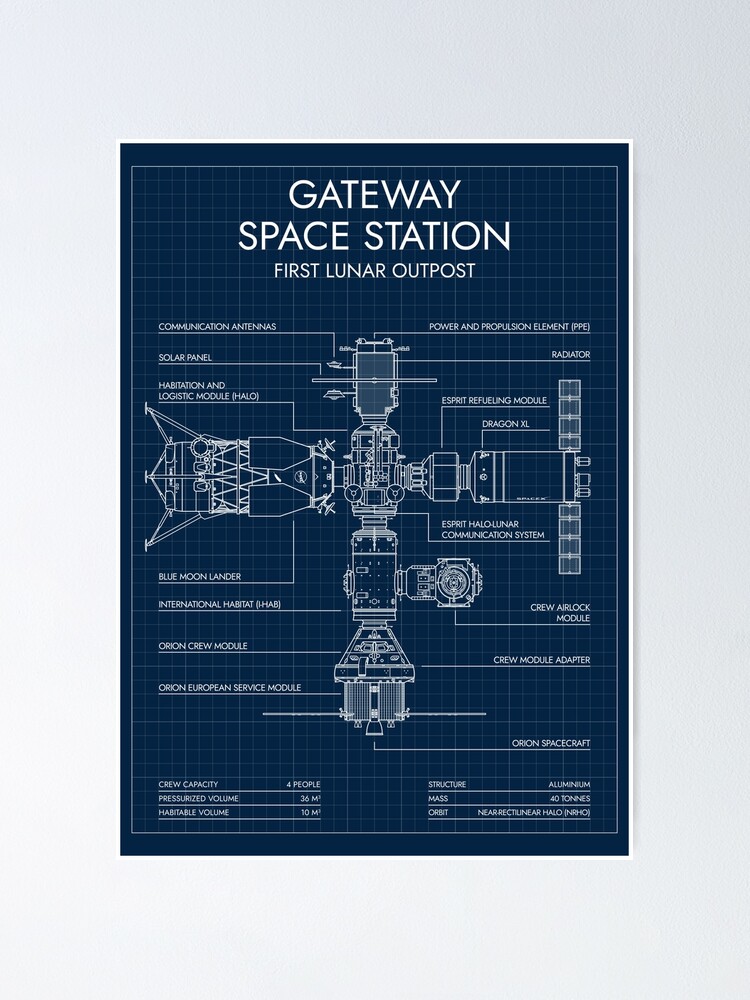The pamphlet titled "Gateway Space Station: First Lunar Outpost" features a detailed blueprint of a space station or satellite against a dark blue background with a white grid overlay. The title is prominently displayed in white text at the top. The blueprint itself is a segmented, vertical diagram of the space station, meticulously labeled. Key features identified include "Communication Antenna," "Solar Panel," "Power and Propulsion Element," "Hydration and Logistical Module," "Halo Lunar Communication System," "Radiator," "ESPRI Refueling Module," and "DragonXL." These labels are connected with lines to their respective parts, allowing for easy identification. Additional specifications, such as "Structure Aluminum Mass: 40 tons," are noted towards the bottom of the diagram, providing further technical details about the space station's design and components.